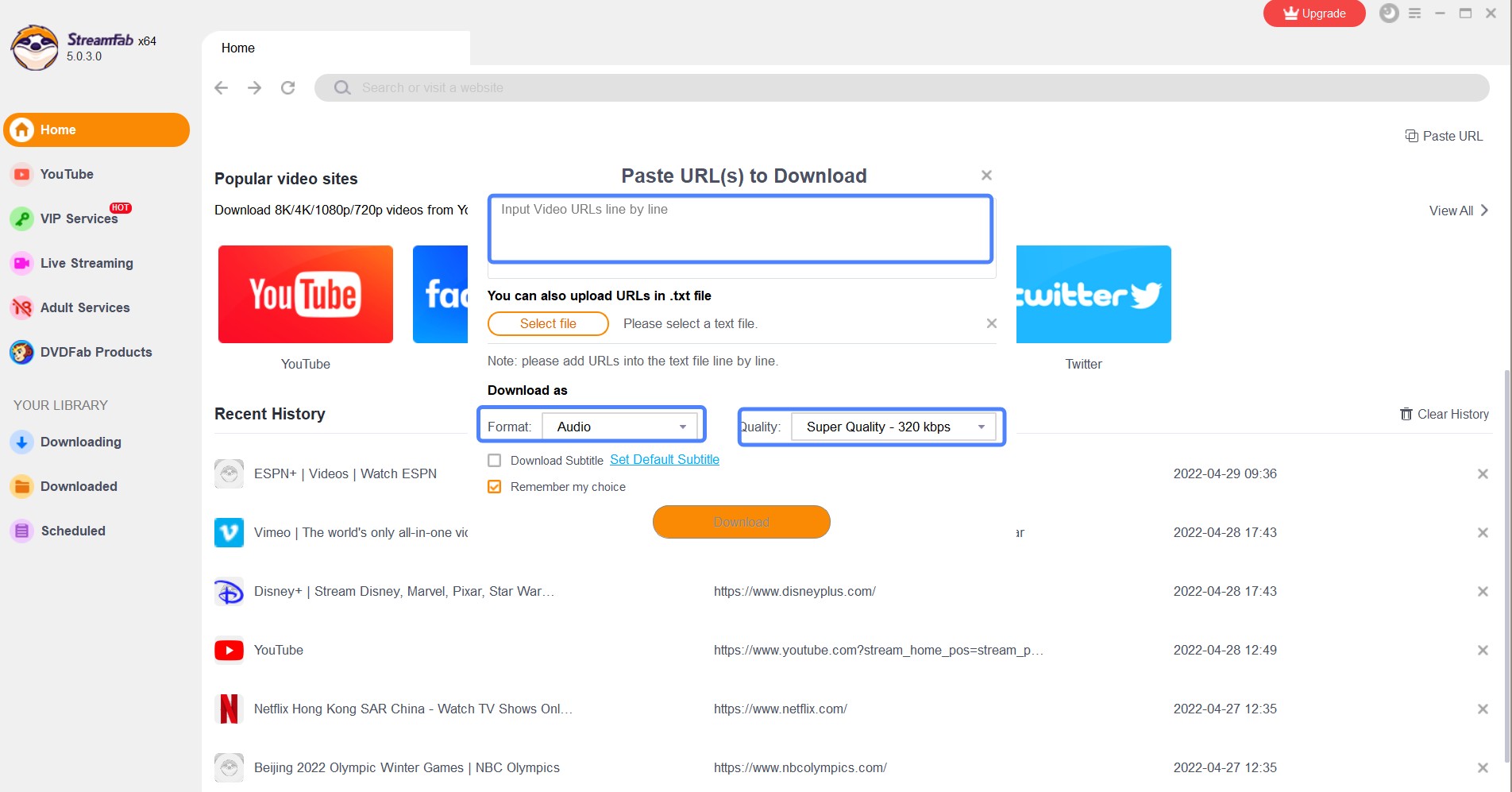### Detailed Caption for StreamFab Application Screenshot

The screenshot showcases an application called **StreamFab**, prominently displaying the label "StreamFab X64" in the upper left corner, indicating the version as 5.0.3. The application's logo, a small, cartoonish furry animal, is encased in a gray border, adding a whimsical touch to the otherwise functional interface.

Immediately beneath the logo, the left-hand sidebar lists several categories:
- **Home** (highlighted with an orange rectangular oval, suggesting it's the currently selected option)
- **YouTube** (marked with a traditional red and white play button)
- **VIP Services** (represented by a key icon)
- **Live Streaming** (depicted with a camera icon)
- **Adult Services**
- **DVDFab Products**

Below these categories lies a section titled **Your Library**, which includes subsections for **Downloading**, **Downloaded**, and **Schedule** — each having relevant icons next to them.

The main content area features a field labeled "Popular video sites," accompanied by instructions to paste URLs for downloading videos. It suggests compatibility with platforms like YouTube, Facebook, and Twitter, inferred from the icons arrayed around the URL input box. At this moment, no URL is pasted.

Additional settings for downloads are shown:
- **Format**: Audio
- **Quality**: Super Quality

At the bottom, a section titled **Recent History** lists previously downloaded content with thumbnails, titles, sources, and download dates (all from 2022). Some of the entries include:
- ESPN videos
- A video from Vimeo titled "the world's only…" (partially cut off)
- Disney Stream, with the Disney website indicated
- YouTube
- Netflix
- Content from Hong Kong SAR, China
- Beijing 2022 Olympic Winter Games

The organized layout, combined with visually distinct icons and highlights, suggests that StreamFab is a robust tool designed for downloading video streams from multiple popular platforms.